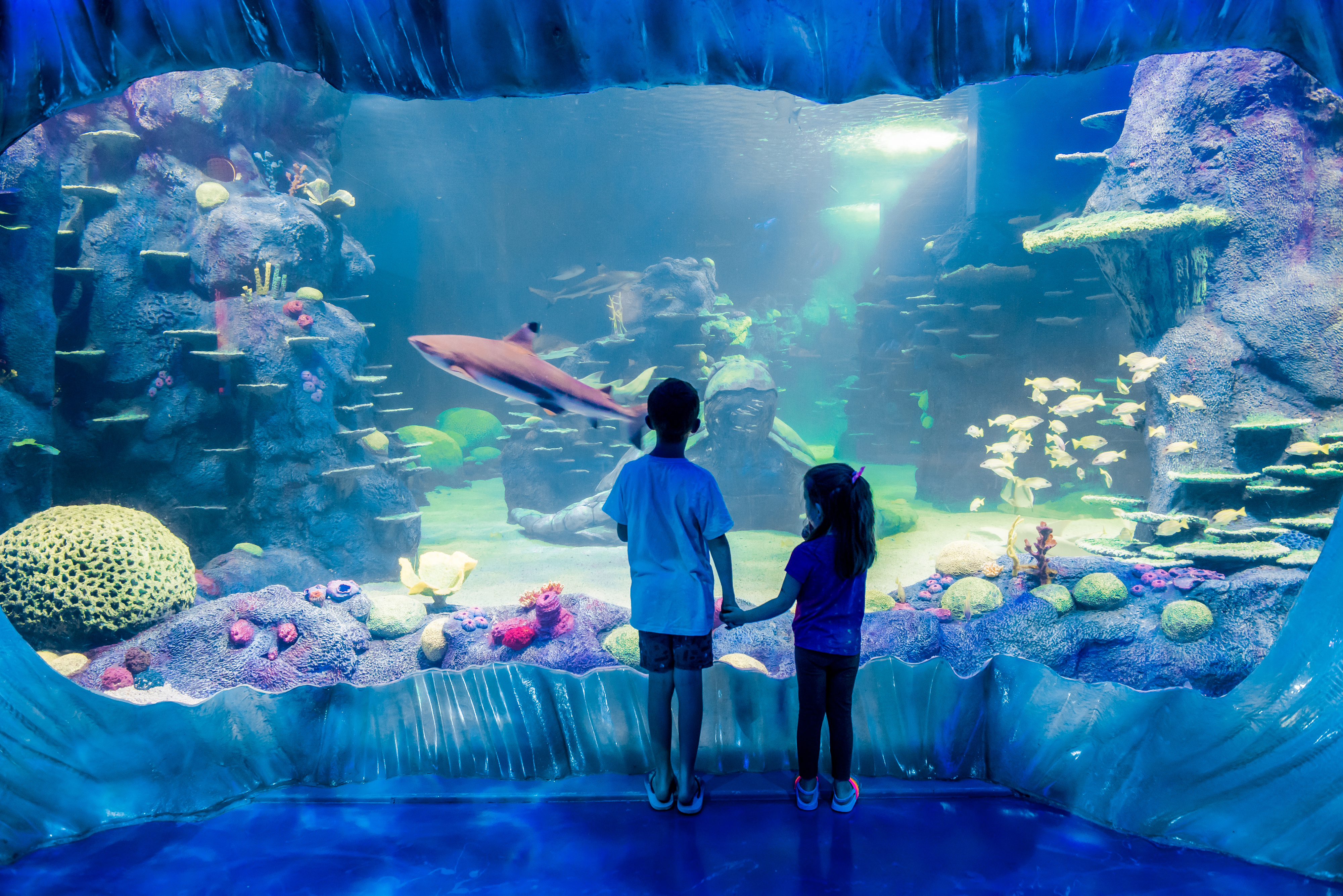In this captivating image, two young children, presumably a brother and sister, stand hand-in-hand with their backs to the viewer, gazing at a mesmerizing aquarium. The boy, about eight years old, sports a white t-shirt, surf trunks, and flip-flops, while his little sister, around four years old, wears a purple shirt, black pants, and white flip-flops, her long black hair tied back with a pink hair tie. They stand on a shimmering blue floor designed to mimic the appearance of ice or water, within an environment crafted to immerse visitors in an undersea world. To their left, a large gray shark glides regally through the water, accompanied by another shark barely visible in the background. The right side of the tank teems with a lively school of yellow fish. The aquarium is intricately decorated with realistic coral and rock formations, enhancing the illusion that the children are inside the watery habitat alongside the marine creatures. Light filters through the blue water from above, illuminating the scene and captivating the children's imaginations.